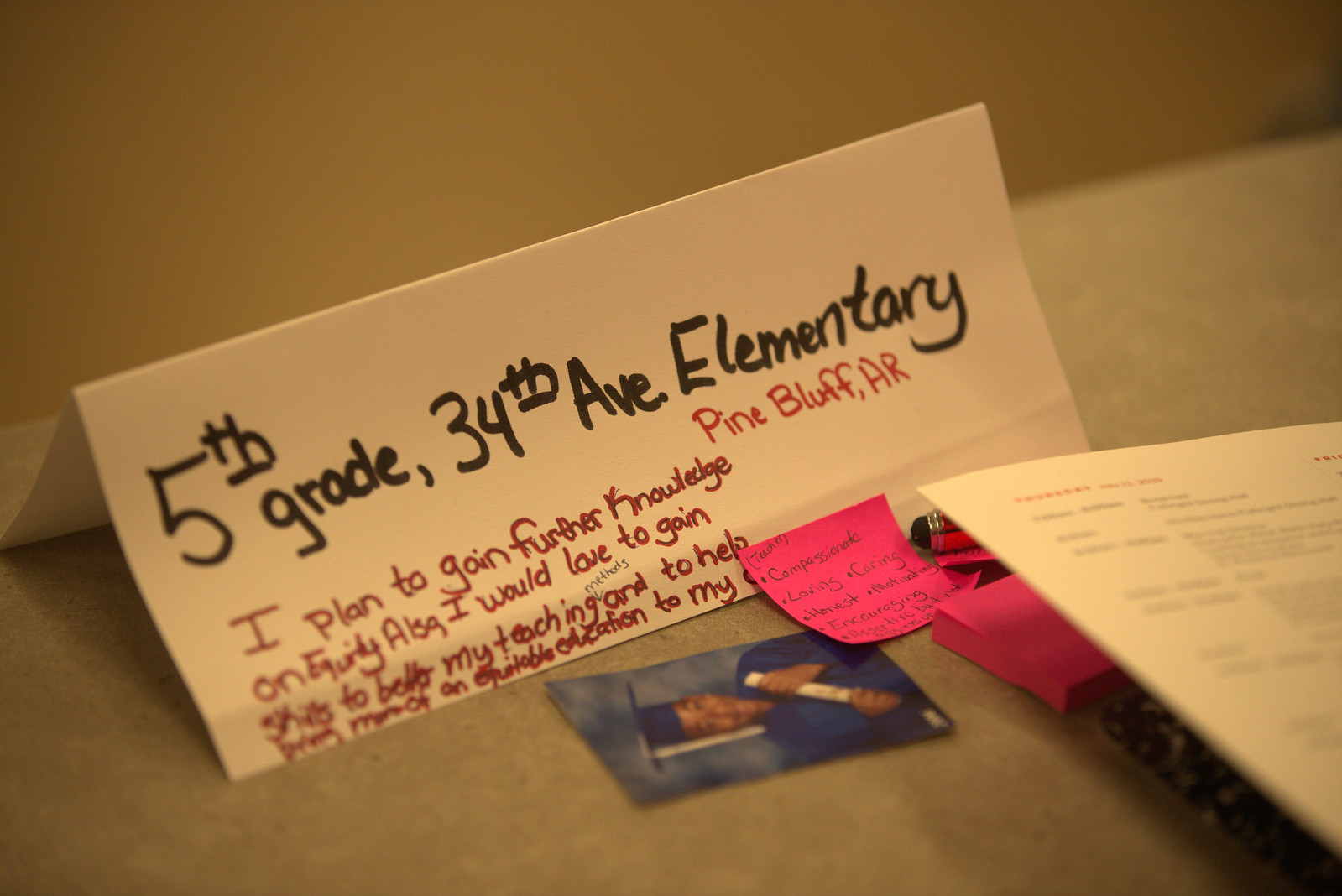The image depicts a stonetop desk right against a beige-colored wall under dim lighting. On the desk, a piece of white paper is folded in half and propped upright in a triangular shape, functioning like a sign. The paper features prominent black marker text stating "Fifth Grade, 34th Avenue Elementary" and in red, "Pine Bluff, AR." The text continues at the bottom left, though partially blurry, expressing a commitment to gaining further knowledge on equity and teaching skills to promote equitable education.

In front of the paper sign, there is a photograph of a young black child dressed in a blue graduation cap and gown, holding a diploma. To the left, there is a pile of papers with a pink Post-it note listing traits such as "Compassionate, Loving, Caring, Honest, Motivating, Encouraging, Assertive but not Aggressive." Additionally, a book is slightly visible in the bottom right corner of the image, though the details are blurry.